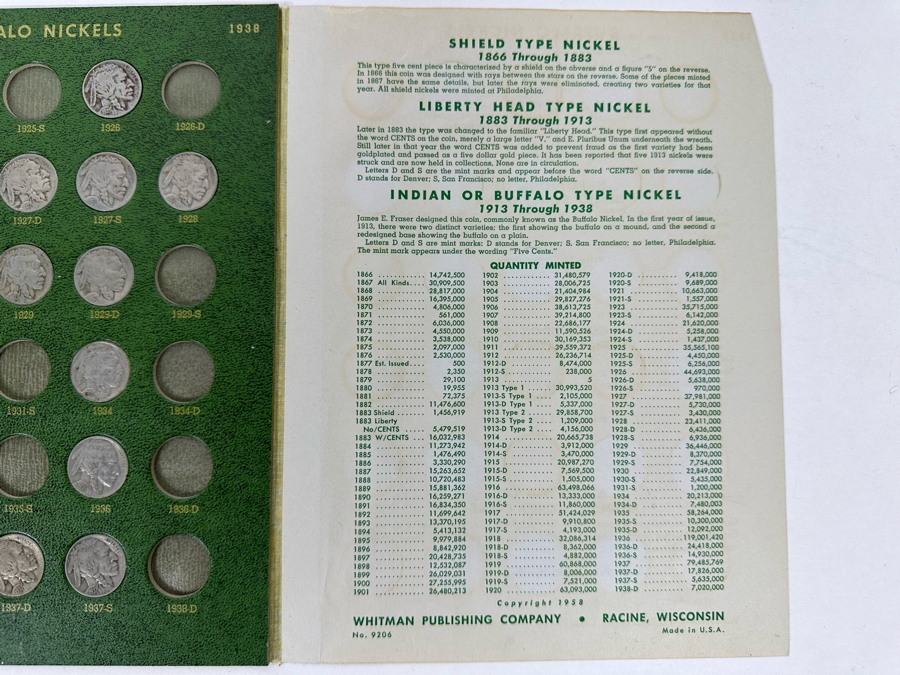This photograph showcases an intriguing coin collector's book, primarily dedicated to Buffalo nickels, spanning from 1913 to 1938. The left half of the image displays a green cardboard backing with meticulously cut out slots, some filled with nickels, organized by year and mint mark (S, D, or no mark). The heading "Buffalo Nickels 1938" is cut off at the top, and beneath it, each slot indicates the specific year the nickels were minted. 

Adjacent to this, the right half of the page is white, featuring informative green text. It highlights three types of nickels: "Shield Type Nickel 1866-1883," "Liberty Head Type Nickel 1883-1913," and "Indian or Buffalo Type Nickels 1913-1938," each accompanied by descriptive paragraphs. Further down, a detailed table lists the quantity minted for each year, differentiated by mint mark. At the bottom of this page, it states the publisher information: "Whitman Publishing Company, Racine, Wisconsin, Number 9206, Made in USA." The book is an illustrative and historical catalog, showing both the years of minting and the production quantities, making it a valuable resource for coin enthusiasts.